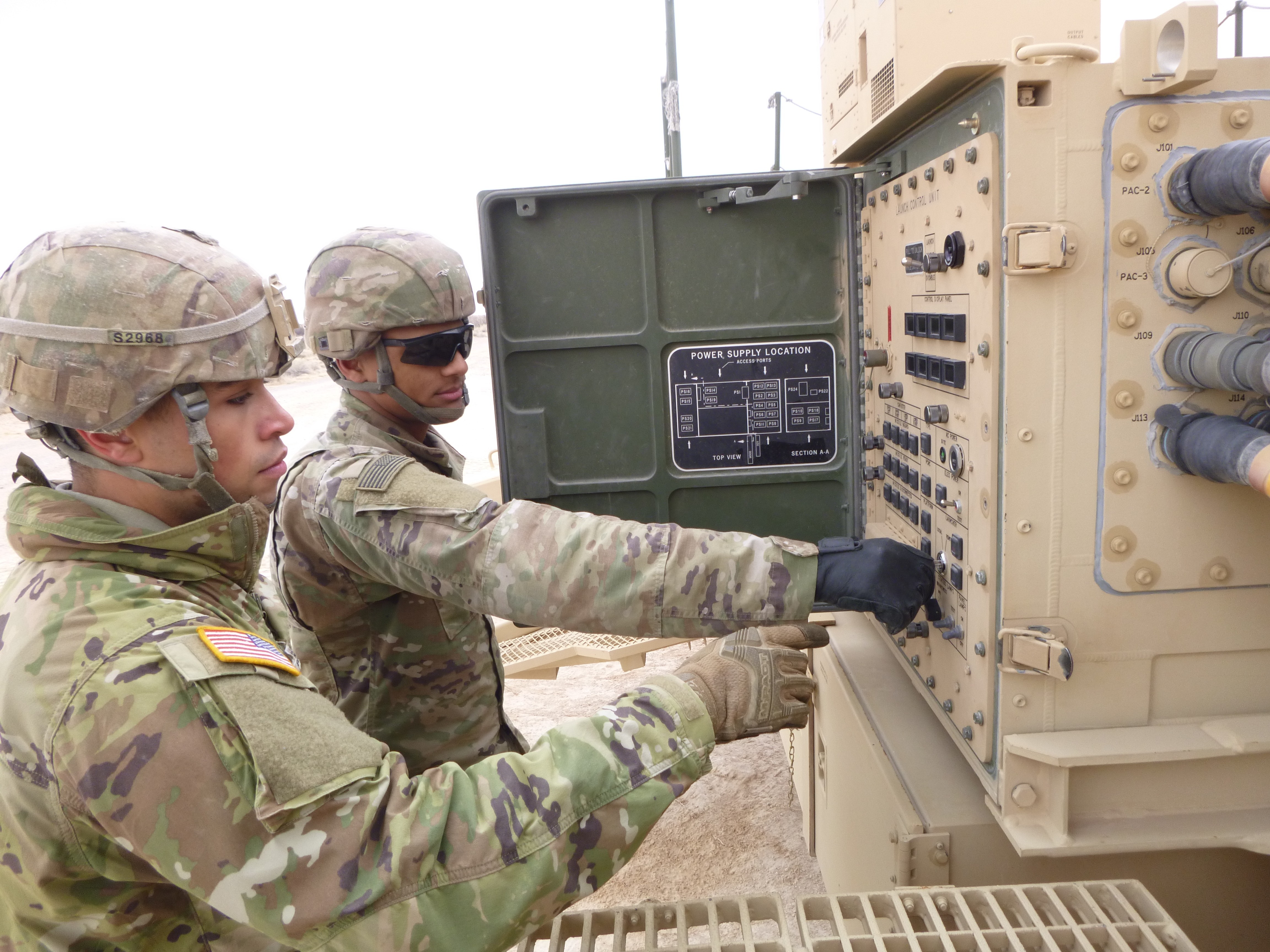In this detailed image, two men are depicted in full army camouflage attire, including jackets, gloves, and helmets marked with numbers, one reading S-2968. One man wears sunglasses, and the other does not. They are working at a large, beige-toned control panel, potentially mounted at the back of a military truck, visible with its open door, displaying an army green interior. The control panel is equipped with numerous buttons, switches, and knobs, and several gray and tan hoses labeled PAC-2, PAC-3, J-109, and J-113, extending from its side. One man is actively pressing or turning the buttons while the other points at them. The men stand on a dirt road, and the scene seems to be outdoors, with some additional metallic structures visible in the background. The man on the right also sports an American flag patch on his uniform's shoulder.